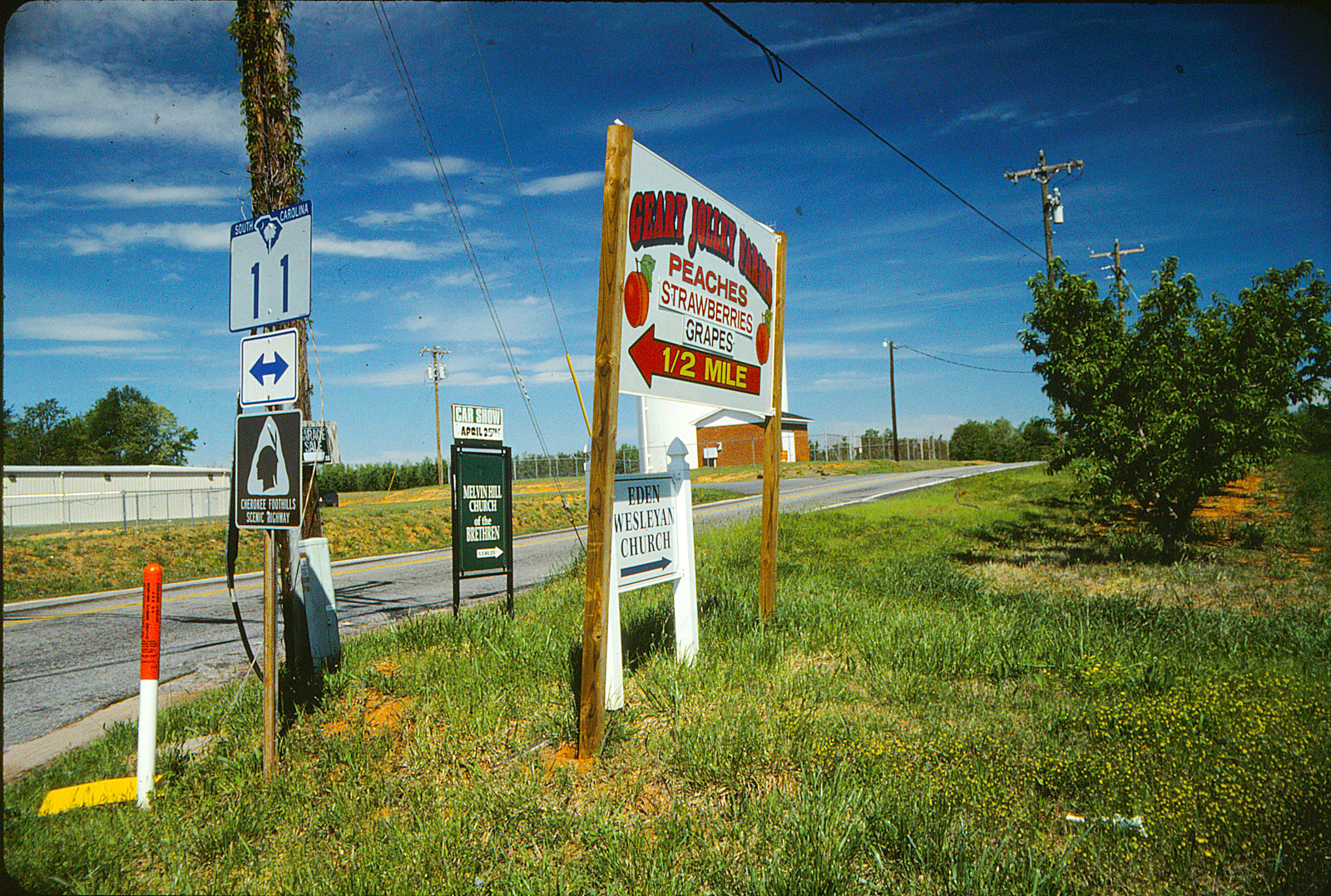A daytime photograph captures a street corner where a mix of green and dead grass surrounds the area. A road starts from the bottom left of the image, running vertically and veering slightly to the right. Prominently, there's a sign supported by two wooden fence posts, featuring a white background with red lettering. The sign advertises peaches and strawberries with a large red arrow pointing left, indicating a distance of one-half mile in yellow lettering. A telephone pole stands to the left of the sign, with wires extending to the right and connecting to additional poles. On the left side, a pavement road is visible. To the right, the area is flanked by trees, possibly apple orchards. A small red and white post is positioned in the bottom left corner. Below the primary sign, there's an additional white sign. The sky is blue with scattered clouds, adding to the serene atmosphere. Across the street, a white building sits on the left side of the image, and a brown building is visible in the distant background.